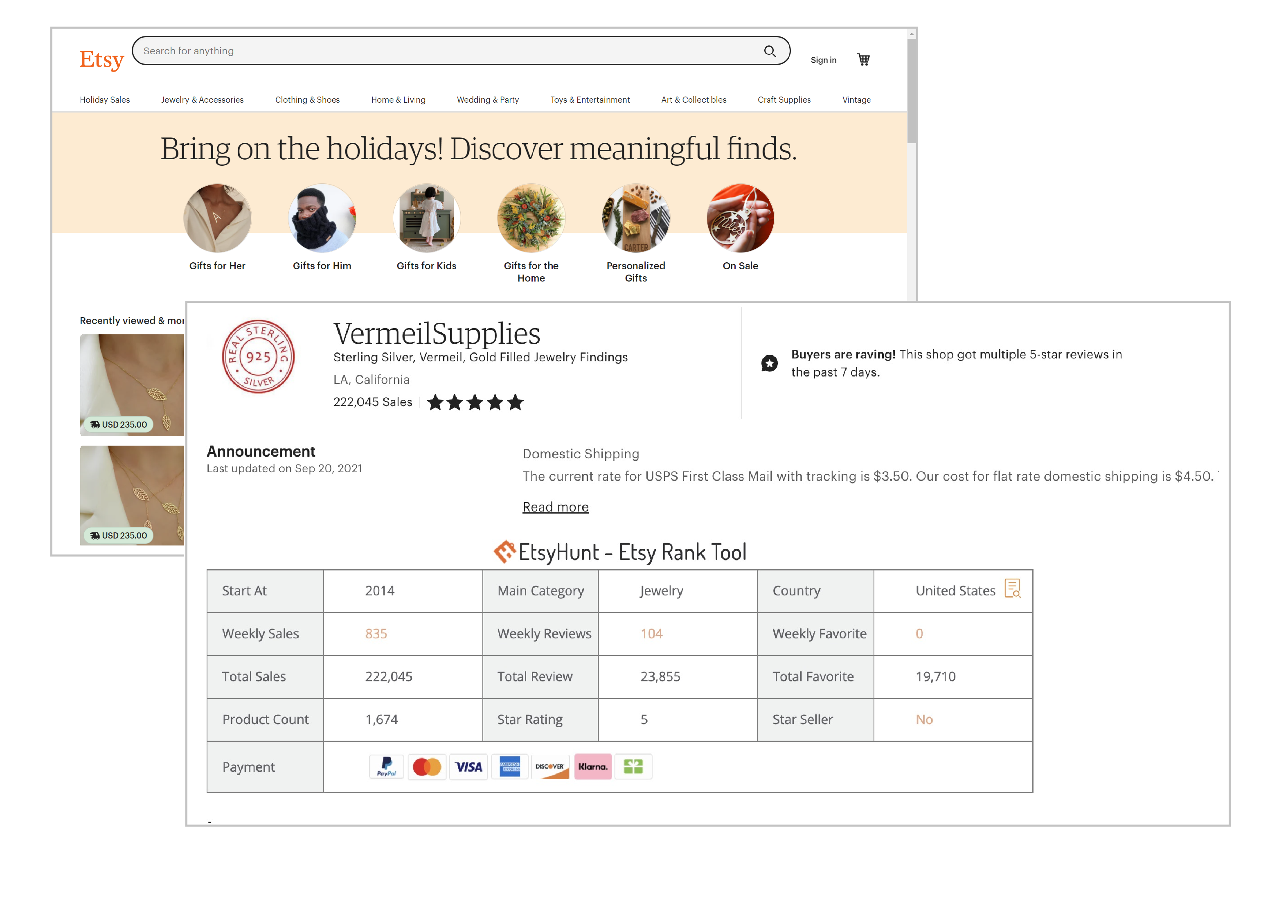The image depicts the homepage of the Etsy website. The Etsy logo, prominently displayed in orange, sits at the top left corner. Adjacent to the logo is a search bar icon marked with "MT". The main banner is eye-catching, featuring the tagline "Spring into the holidays. Discover meaningful finds," displayed in large, readable text.

Below the banner, six circular icons serve as categories for browsing: "Gifts for Her," "Gifts for Him," "Gifts for Kids," "Gifts for the Home," "Personalized Gifts," and an unspecified category likely meant to direct users to different sections of the site for easier navigation.

Further down, there is a section labeled "Recently viewed," showcasing an image of a woman's neck adorned with a necklace. The image appears twice within a square box format. The central text reads, "Vermeil Supplies, Sterling Silver, Vermeil, Gold Filled Jewelry Findings," accompanied by a five-star rating, indicating high customer satisfaction.

The structured layout and vivid details are carefully curated to enhance user experience, helping visitors easily find and explore various gift options on the platform.